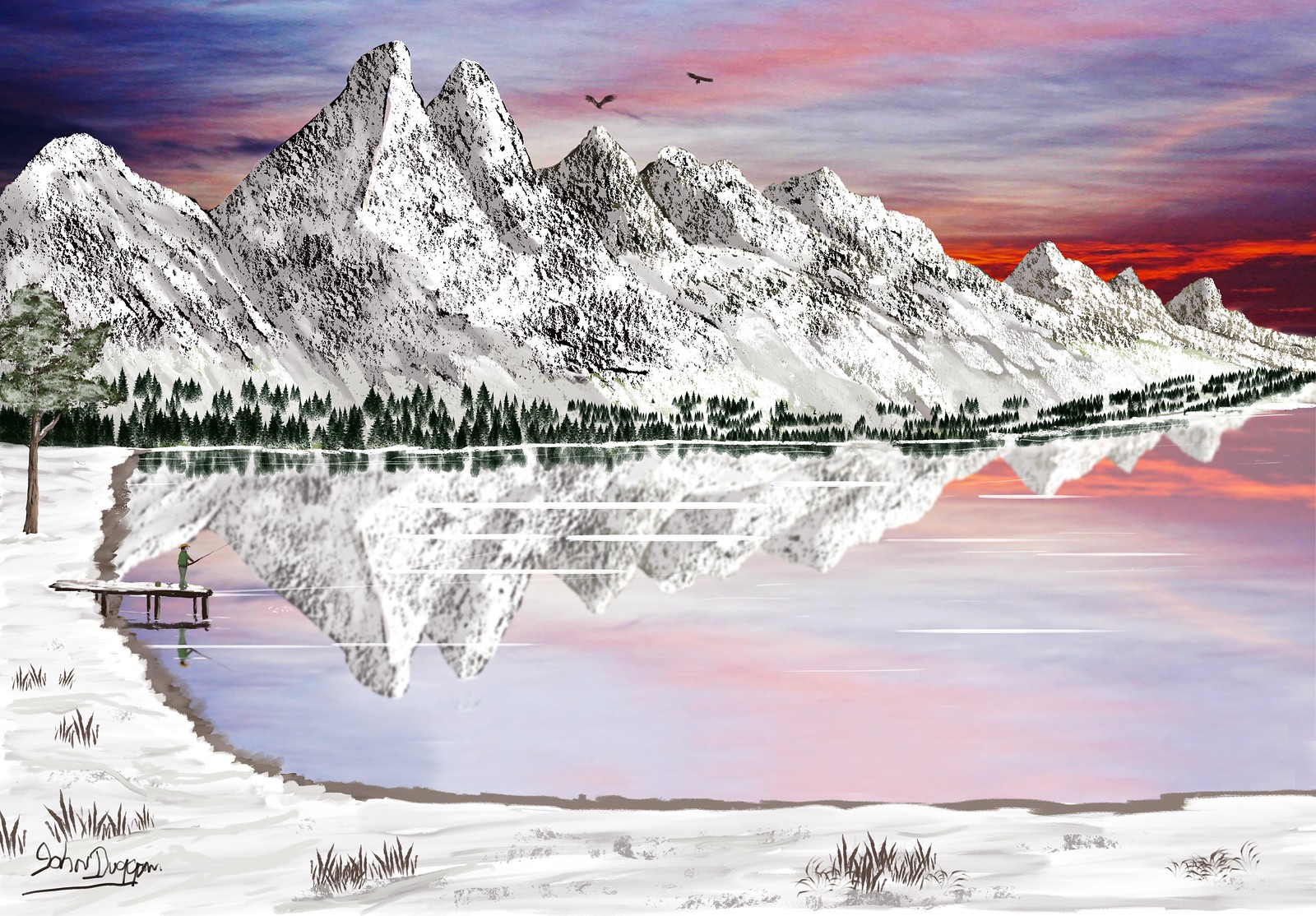This intricate digital artwork depicts a serene snowy landscape bathed in the final hues of sunset. The sky displays a vivid dance of red, purple, pink, and dark blue, casting a dramatic ambiance over the scene. Dominating the upper portion of the frame, a majestic range of snow-capped mountains stands imposingly. Above these peaks, a couple of birds soar gracefully, adding a touch of life to the remote wilderness. At the base of the mountains, a ridgeline adorned with clusters of small pine trees slowly transitions to a tranquil lake below. The lake's surface mirrors the stunning mountain range and vibrant sky with near-perfect clarity, enhancing the overall sense of calm and symmetry. To the left side of the frame, a solitary man fishes quietly from a small pier, completing the picturesque scene with a touch of human presence.